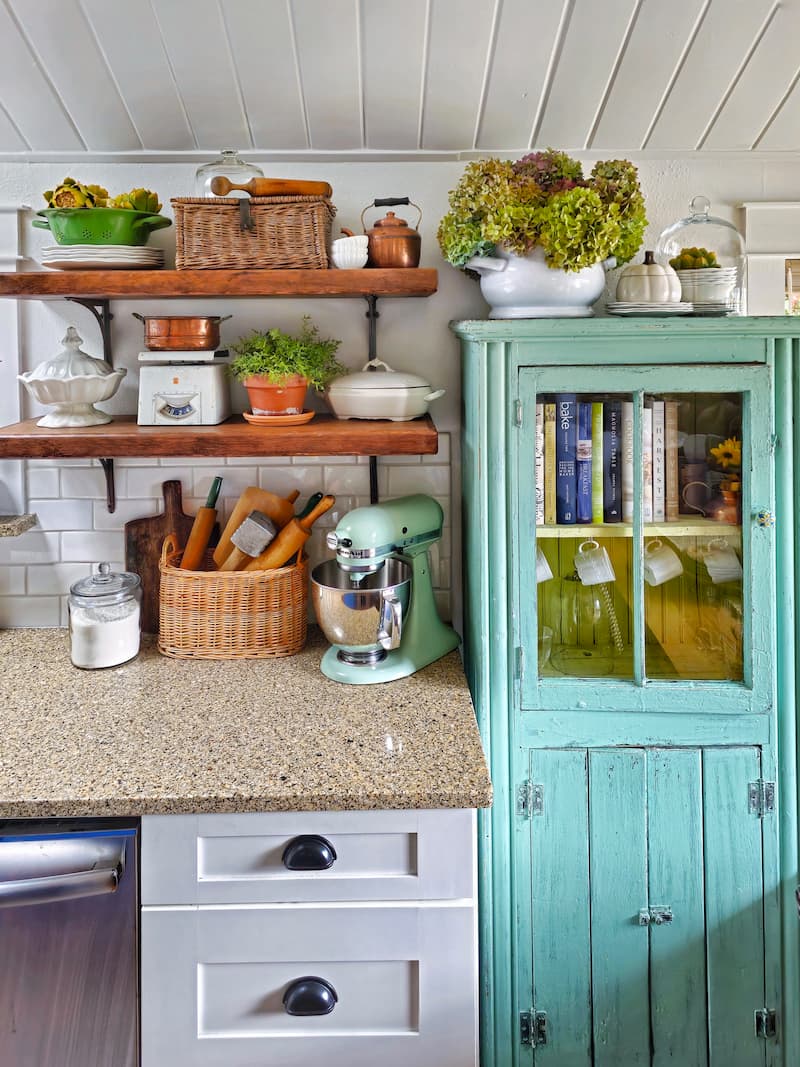This inside picture captures a detailed view of a cozy, vintage-style kitchen corner. The ceiling consists of white wooden boards, complementing the white walls. Dominating the far right is a turquoise aqua-colored cabinet with a glass front, showcasing a collection of cookbooks on the top shelf and hanging coffee cups along with other dishes on the lower shelf, though the latter is shadowed and indistinct. Below, it features an accessible cabinet space with black handles.

Adjacent to this cabinet are a series of brown shelves adorned with various antique and practical kitchen items. These include a wicker basket, a food scale with a copper top and white base, a white candy dish, and a vibrant house plant. A glass dish filled with sugar sits next to another wicker basket holding rolling pins and additional kitchen utensils. Nearby, a stylish turquoise KitchenAid mixer with a silver bowl rests on a brown and beige-spotted desk-like surface, complementing the white cabinet beneath it that has black knobs.

Adding to the charm, a small shelf holds a green bowl filled with fruit atop some white plates, another wicker basket with a wooden spoon, a copper tea kettle with a black handle, and several more decorative items like a white candy dish, a small decorative box with a copper pot atop it, and additional bowls.

This kitchen corner is not only aesthetically pleasing with its vintage and antique elements but also brimming with practical kitchen tools and cozy décor.